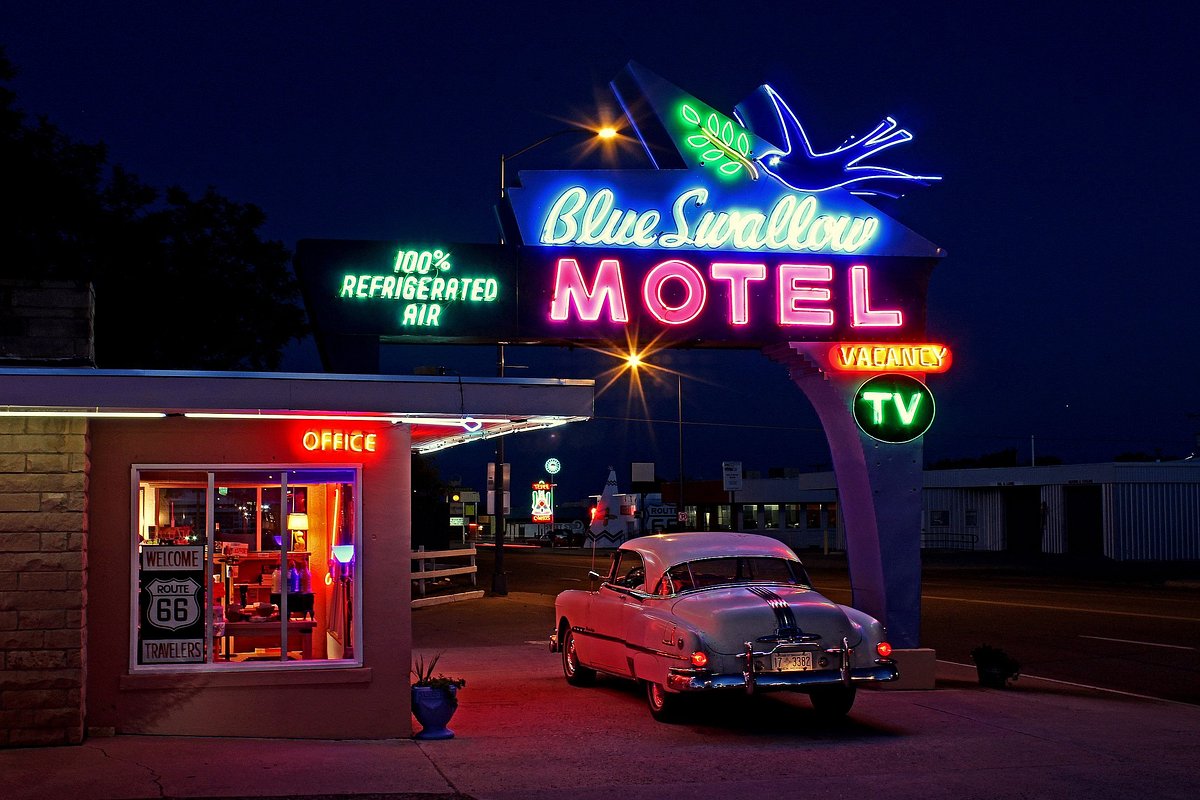This detailed digital rendering captures the nostalgic charm of a vintage 1950s motel called the Blue Swallow Motel. The scene is set at night, illuminated by vibrant neon lights. At the center, the prominent motel sign reads "Blue Swallow Motel," with "Blue Swallow" in blue and white lettering and "Motel" in pink. A blue bird carrying a green branch is depicted above the text. To the right of the main sign, additional signage reads "Vacancy" in red, and a black circle below it features "TV" in green text.

Beneath the sign, an old 1950s car is parked, characterized by its roundish features and pink hue, with the license plate 1733H2 visible. On the far left, the motel office is housed in a brick building, identified by a red LED "Office" sign. Above the entrance, green neon letters advertise "100% Refrigerated Air." A window in the office features a welcome sign reading "Welcome to Route 66," and a potted plant adorns the exterior. The right side of the scene is shrouded in darkness, hinting at other buildings without revealing their details.

Overall, this image beautifully encapsulates the retro ambiance of a classic American motel along the historic Route 66.